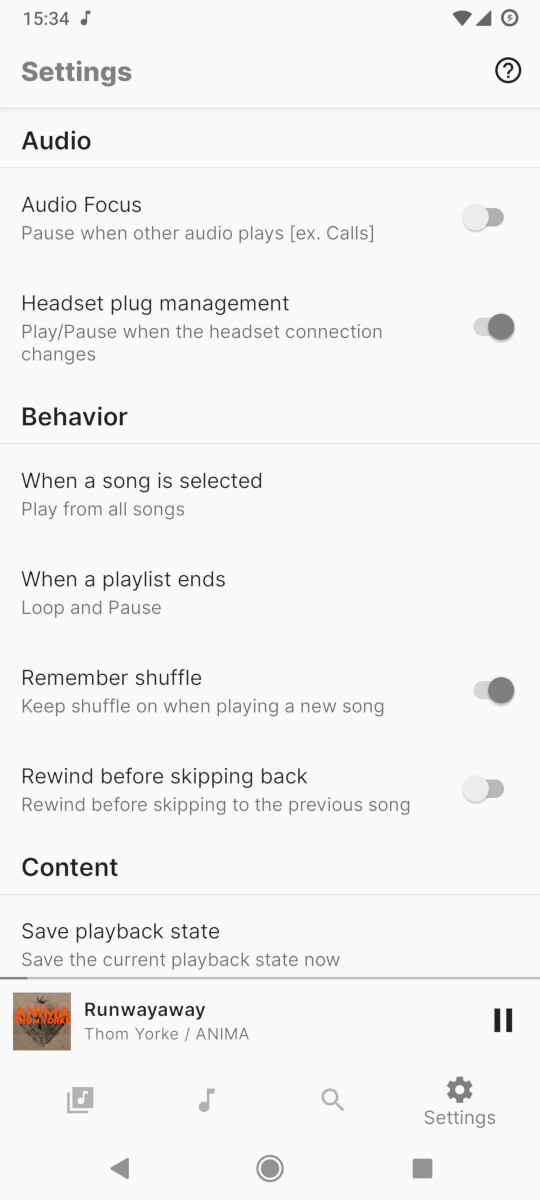The top part of the image shows a smartphone screen with a light gray background and black text. At the very top left corner, the word "Settings" is displayed. Below that, several settings options are listed.

First, there is an "Audio Forecast" setting with a description stating, "Pause when other audio plays (e.g., calls)." The toggle switch for this option is on the right side and is turned off, indicated by a light gray/white color.

Second, there is a "Headset Management" option with the description, "Play or pause when the headset connection changes." This toggle switch is located on the right side and is turned on, indicated by a gray color.

Next, there is a section labeled "Behavior when a song is selected," which includes the following settings:
1. "Play from all song when a playlist ends" has a "loop" and "pause" option. 
2. "Remember shuffle" which is described as "Keep shuffle on when playing a new song," and the toggle switch for this is also on the right side and turned on, marked by a gray color.
3. "Rewind before skipping back" with the description, "Rewind before skipping back to the previous song." The toggle switch for this option is off, indicated by a light gray color and positioned to the left.

Additionally, there is a "Content Save" section with the option to "Save playback state," allowing the user to save the current playback state.

At the bottom of the screen, there is information about the song currently playing, which is "Runaway" by Thom Yorke from the album "Anima." To the right of this information, there is a pause button. Below this, there are icons for settings, search, music, and playlists, all displayed in gray. There is also a logo for the music app, and the text "Anima Runaway" is written in red.